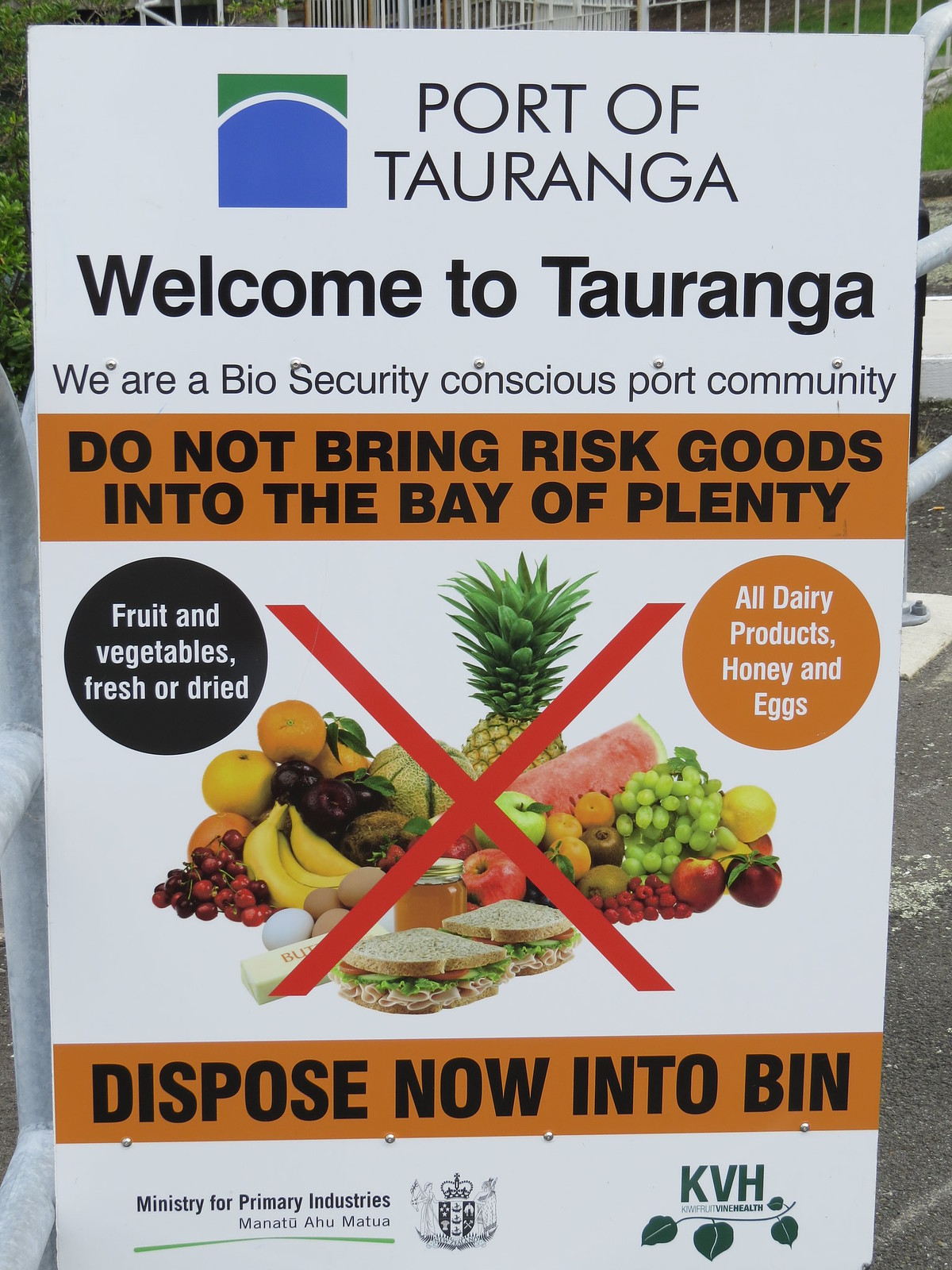The image depicts an informational sign propped up next to a metal gate, characterized by a white background with multiple lines of black text. At the very top in large, bold letters, it reads "Port of Taranga" with an adjacent square featuring an arched blue shape and green top. Below, it states "Welcome to Taranga" followed by the message "We are a biosecurity conscious port community". An orange banner stretches horizontally across the sign, with the stern warning in black text, "Do not bring risk goods into the Bay of Plenty". The lower section resumes the white background, displaying a black circle on the left with white text listing "Fruit and vegetables, fresh or dried" and an orange circle on the right specifying "All dairy products, honey and eggs". Below these circles is an image featuring a variety of prohibited items, including fruits, vegetables, honey, and sandwiches, all marked with a large red X. Beneath the image, in an orange rectangle with black lettering, it urges to "Dispose now into bin". At the bottom left, there is a small text in black, "Ministry for Primary Industries, Manatu Ahumatua", accompanied by a shield symbol or crest to its right.